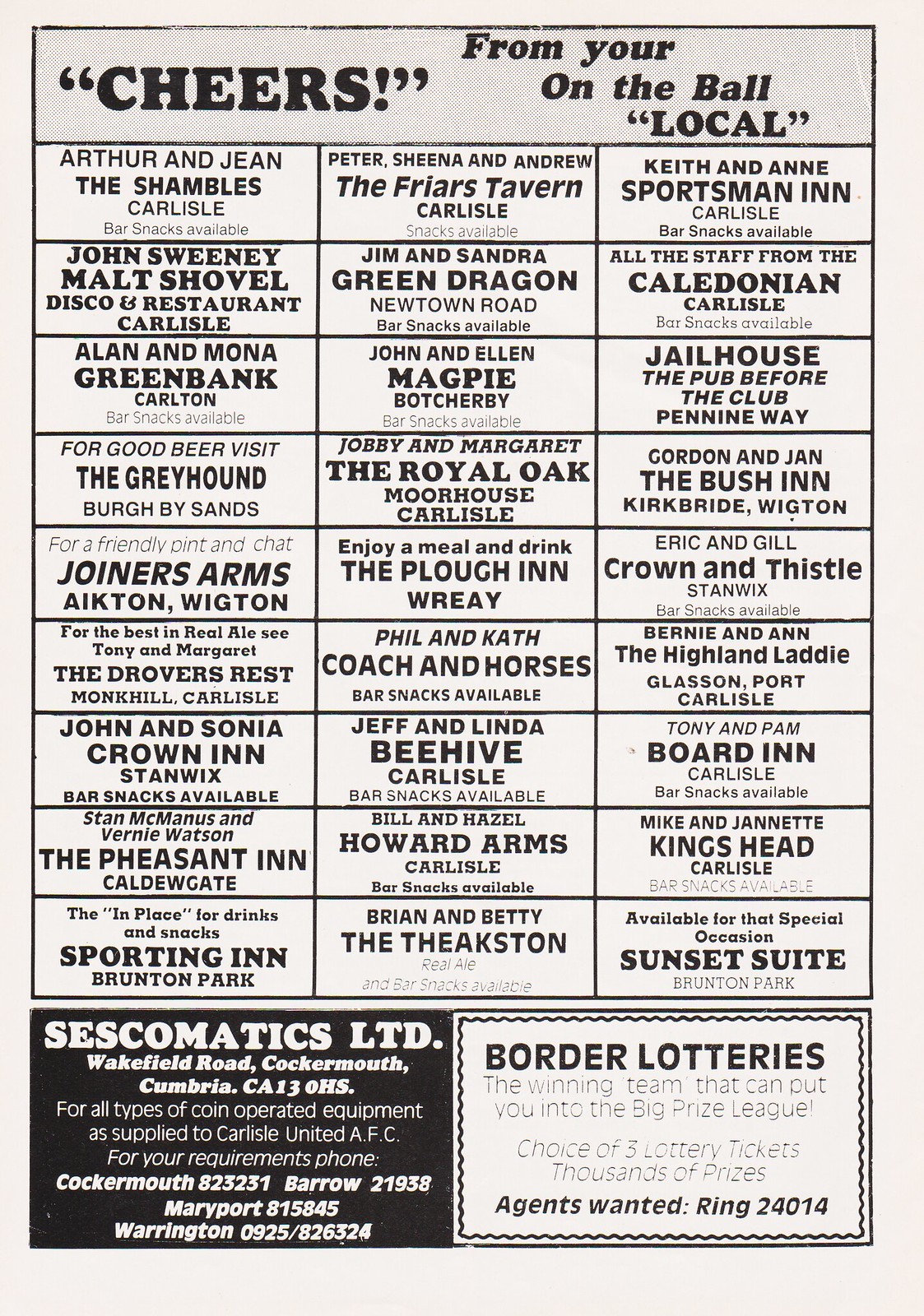The image is a detailed black-and-white flyer filled with advertisements for various local businesses, framed by a border. The top of the flyer prominently displays the title "Cheers from your On The Ball local." The center section of the flyer is divided into multiple black-and-white boxes, each featuring an advertisement for a different establishment, with at least 27 businesses highlighted. These include bars, taverns, inns, and pubs such as The Friars Tavern, Sportsman's, Jailhouse, The Pub Before The Club, Penway, Green Dragon, The Board Inn, Kingshead, and Sunset Suites. Each advertisement lists the establishment's name along with the owner's names and sometimes additional details, such as "bar snacks available" and "for good beer visit the Greyhound Berg by Sands." The flyer also mentions specific locations like Carlisle, Kirkbridge, Wiginton, and Brunton Park. At the bottom, there are two additional advertisements: one for Sescomatics Limited, which supplies coin-operated equipment to Carlisle United AFC, and another for Barter Lotteries, promoting their big prize league.